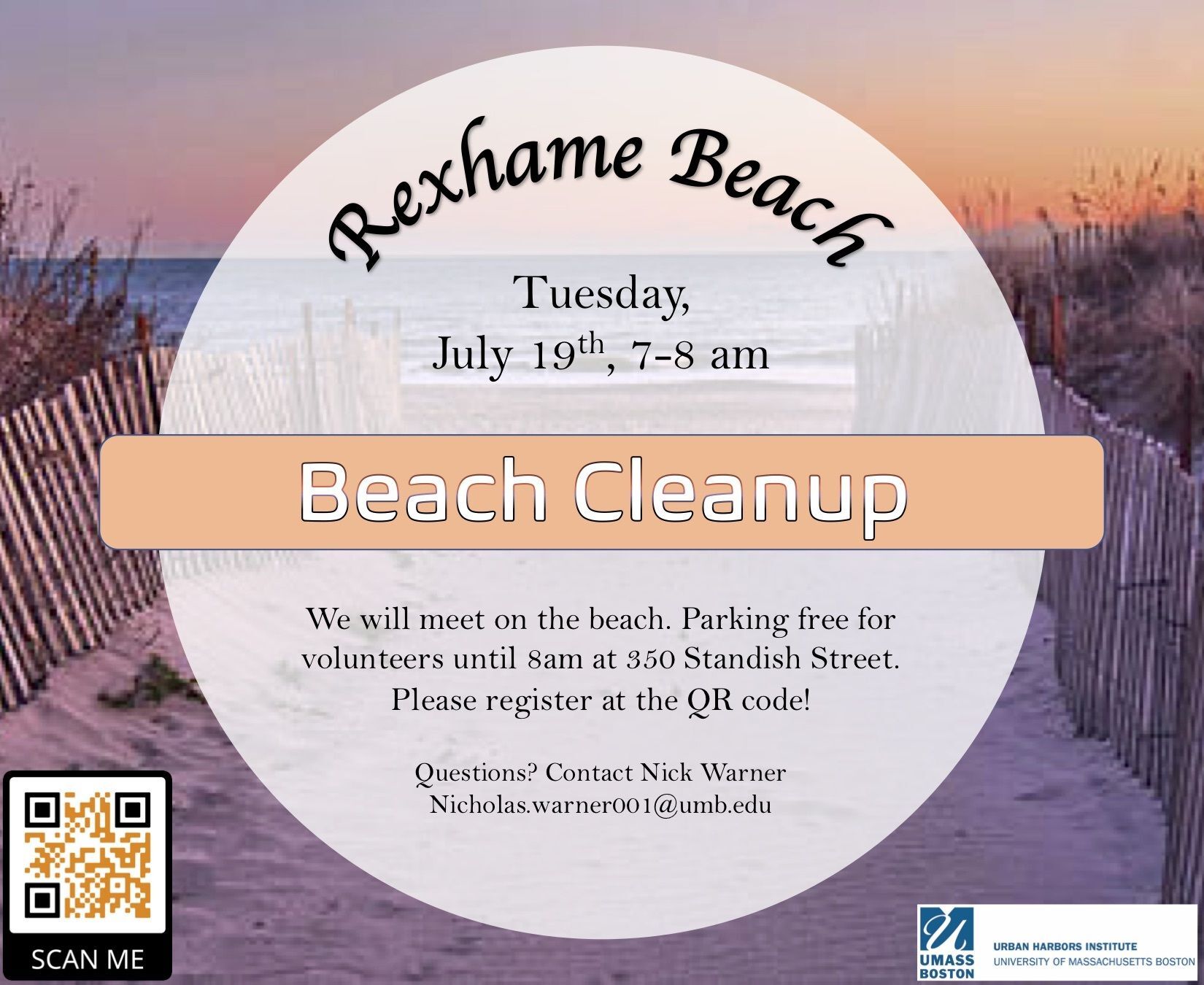The image is a detailed poster for a beach cleanup event. The background features a vibrant sunset sky with hues of blues and pinks over the ocean, and a sandy beach path leading towards the water, bordered by a wooden fence on either side with vegetation in shades of browns and beiges. Central to the design is a large white circle containing essential event information in black text: "Wrexham Beach, Tuesday, July 19th, 7 to 8 a.m. Beach Cleanup." Below this, it states, "We will meet on the beach," and mentions free parking for volunteers until 8 a.m. at 350 Standish Street. Volunteers are encouraged to register via a QR code situated in the lower left corner, which reads "Scan me." For further inquiries, the contact email provided is "Nicholas.warner001@umb.edu." In the lower right corner, the poster highlights sponsors, including "UMass Boston, Urban Harbors Institute, University of Massachusetts, Boston."